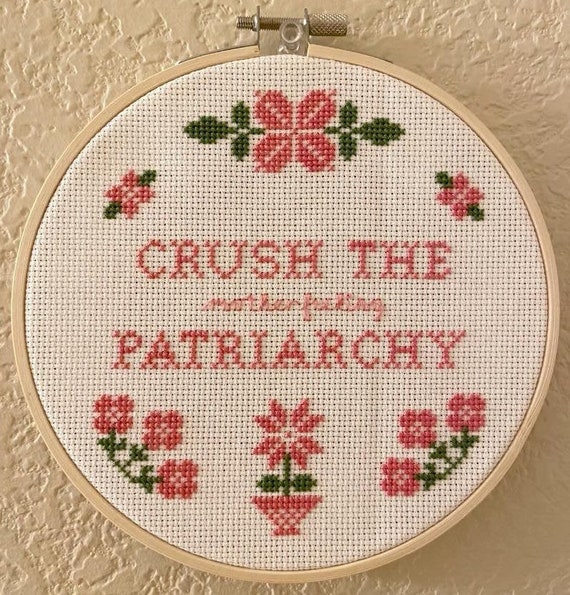The image features a round embroidery hoop that holds a piece of embroidery with a white background. Encircling the center are various types of pink flowers, interspersed with green leaves, arranged decoratively at the top and bottom. Central to the embroidery is the bold and provocative phrase, "Crush the motherfucking patriarchy," stitched prominently in pink thread. This juxtaposition of traditional, delicate needlework with a rebellious message creates a striking contrast. The embroidery appears to be mounted on a beige, stucco-style wall, possibly displayed as a decorative piece. The detailed needlework and the contemporary statement suggest it could be a personal, hand-made project reflective of modern sentiments.